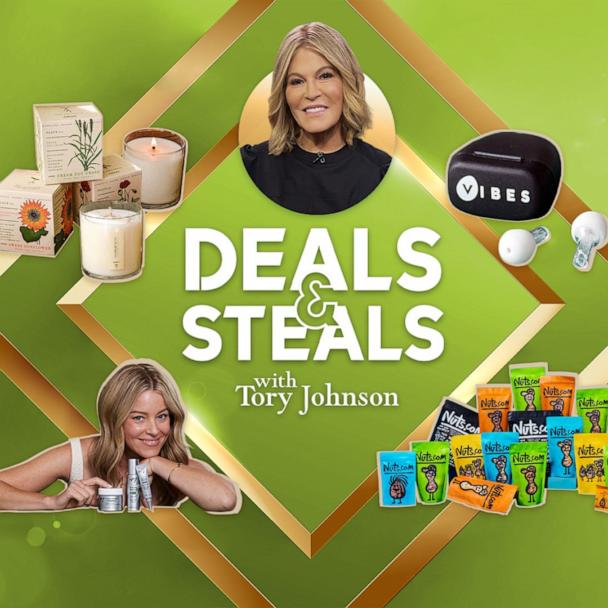This advertisement promotes the show "Deals and Steals with Tori Johnson." At the center of the image is the show's logo, displaying the title "Deals and Steals with Tori Johnson" in bold letters, enclosed within a gold-bordered diamond shape against a green and grey background. Above the logo, there's a smiling graphic of Tori Johnson, whose head slightly extends above the diamond to capture attention. Surrounding the logo, the background features two gold triangles of different sizes. In the top left, there are boxed and unboxed candles, suggestive of sustainable products with floral and grass designs. To the right of Tori’s graphic, there are earbuds branded "Vibes" in a black case. In the bottom right, various snack bags from Nuts.com are displayed. The captivating arrangement and colorful design make the advertisement eye-catching and informative, though it lacks details on where or how to access the promoted deals.